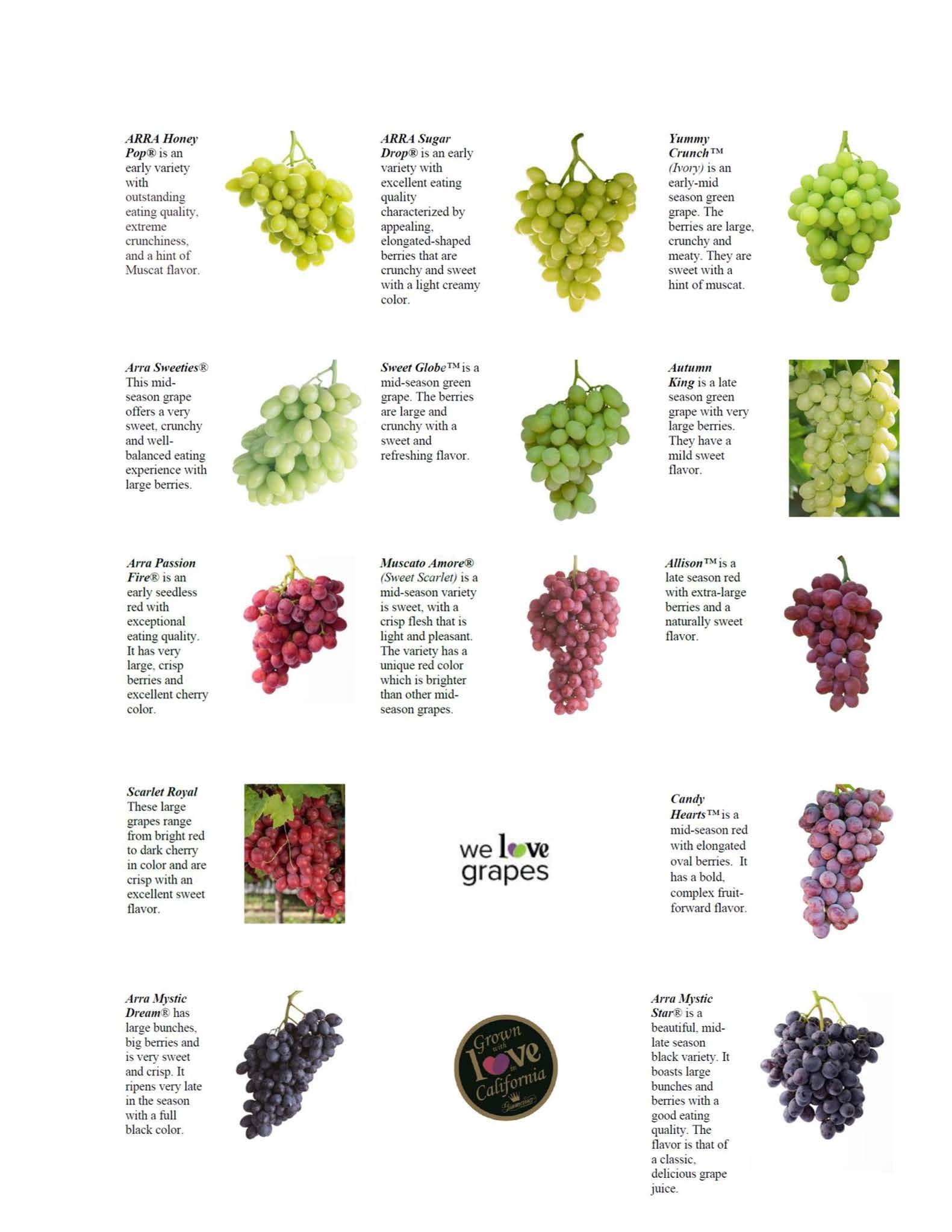The image is a detailed page from a booklet, set against a white background and filled with several small paragraphs of text. Alongside each paragraph, there are vibrant illustrations of various grape varieties. At the top, the text proudly reads "We love grapes," with the "O" cleverly designed as a heart in green and purple hues, reminiscent of grapes. A circular label at the bottom of the page states "Grown with love California," highlighting the origin of the grapes.

Arranged in three columns and five rows, the grapes are categorized by color and variety. The first two rows feature green grapes, ranging from lighter to darker shades. Varieties here include Ara Honey Pop, Ara Sugar Drop, Yummy Crunch, Ara Sweeties, Sweet Globe, and Autumn King. The next two rows showcase red and purple grapes, including Ara Passionfire, Muscat Amore, and Allison. The final row continues with the deeper shades of red and purple, featuring Scarlet Royal, Ara Mystic Dream, Ara Sugar Drop, and Ara Mystic Star.

Each grape variety is accompanied by a descriptive text in black, detailing attributes like taste and texture. For instance, Ara Honey Pop is noted for its outstanding quality and extreme crunchiness with a hint of muscat flavor. In contrast, the Ara Mystic Star is a mid-to-late season black variety known for large bunches and classic delicious grape flavor. Other varieties, such as Allison, are praised for their extra-large berries and naturally sweet flavor, making this image an informative and visually engaging guide to grape varieties.